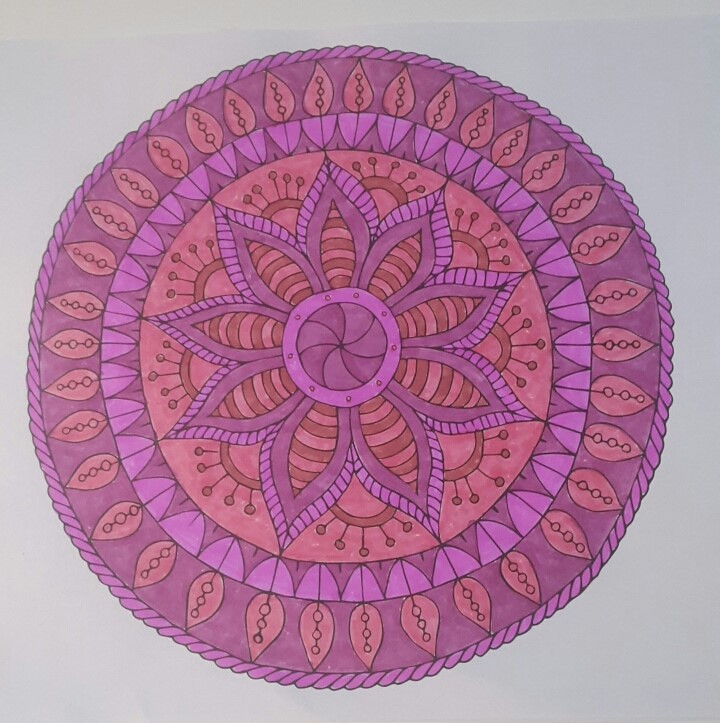The image appears to be a highly detailed piece of textile art or possibly an intricately decorated cloth. The outer edge is bordered by a purple rope-like design, encircling the entire piece. Just inside this boundary lies another purple border adorned with what looks like pink or peach-colored leaves. Further inward, there is a segmented border composed of small purple squares, each featuring dark arrowhead or triangular shapes pointing outward. The central area of the artwork has a pink background with a floral pattern of purple leaves, each outlined with the same rope-like texture, transitioning to a smoother inner border. The centerpiece of the design features a prominent purple flower set against a reddish, floral backdrop, which is intricately detailed with vertigo-like lines and petal motifs extending outward.